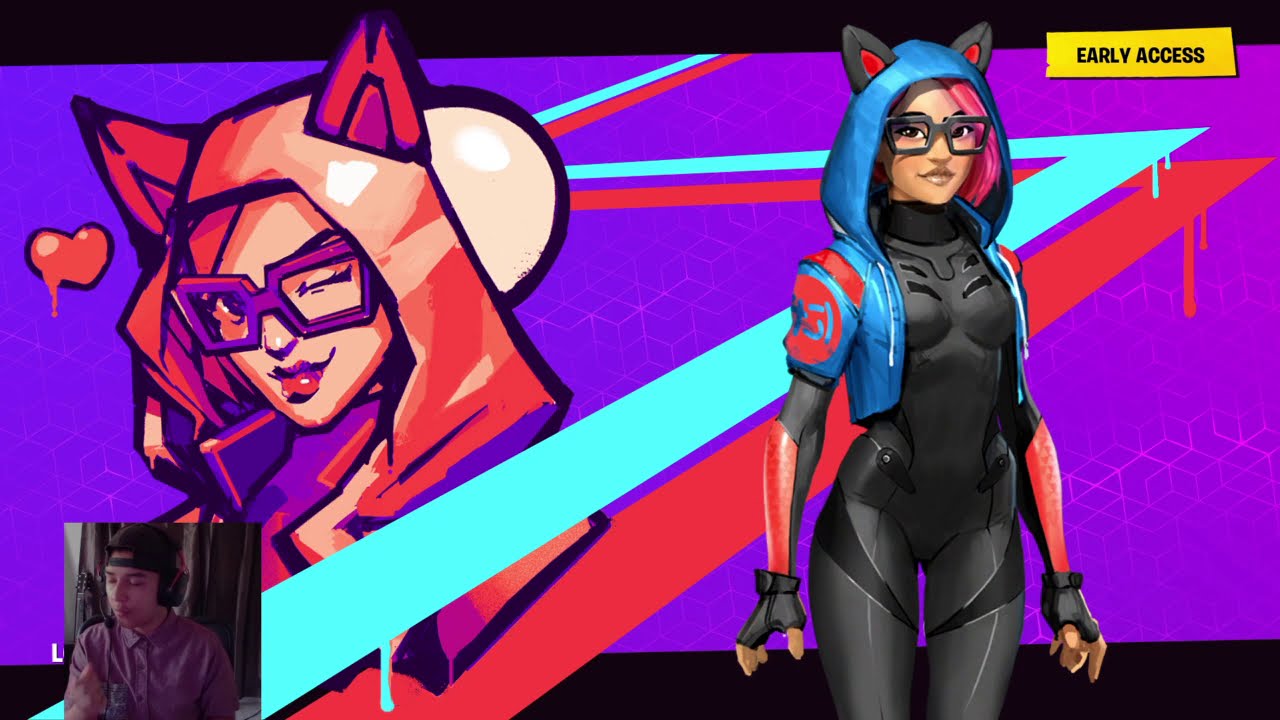The image is a detailed, horizontal screenshot of a game in early access, indicated by a yellow box with the words "early access" in black in the upper right corner. The interface includes a solid black border along the top and bottom edges, framing a vibrant purple background adorned with large, zigzagging blue and red lines that have a dripping effect from their pointed tips. 

Central to the image are two prominent figures. On the right, a female character stands out, wearing a skin-tight black outfit complemented by a blue and red hooded vest. Her attire is accessorized with black gloves that leave her fingers exposed, square black glasses, and black cat ears with red insides protruding from her hood. She has short pink hair and exudes an animated, superhero-like presence. 

To the left, a close-up overlay of the same character is visible, distinguished by a color shift in her hood and vest to pink, rose, and purple hues. This overlay includes a depiction of her with one eye squinted and a small dripping heart to her left, with what looks like the moon in the background.

In the bottom left corner of the screen, a human player, depicted as a teenage boy with a backward ball cap, a button-down shirt, and a microphone-equipped headset, appears to be engaging with the game, possibly commenting or streaming live. The overall aesthetic suggests a mix of manga and modern illustrative styles in a gaming context.